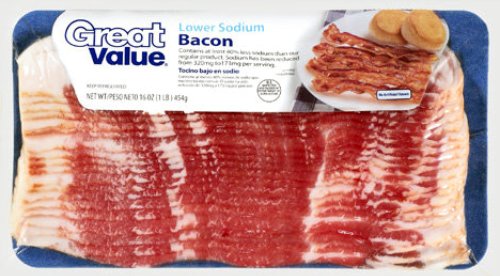This is a close-up, color photograph of a package of Great Value Lower Sodium Bacon, set against a white background. The package features a blue and white tab at the top left where the Great Value logo is displayed. "Lower Sodium" is written in light blue above "Bacon," which is in dark blue text. Directly below this, black text details the ingredients and weight. The bacon itself is raw, displayed against white paper on a blue background. To the right of the label, there is an appetizing image of five to six cooked bacon strips on a plate, accompanied by two biscuits at the top. The bacon in the image appears reddish with white marbling and brown edges, indicating it is cooked. The overall image is cleanly clipped with no jagged edges, suggesting it might be designed for promotional purposes.